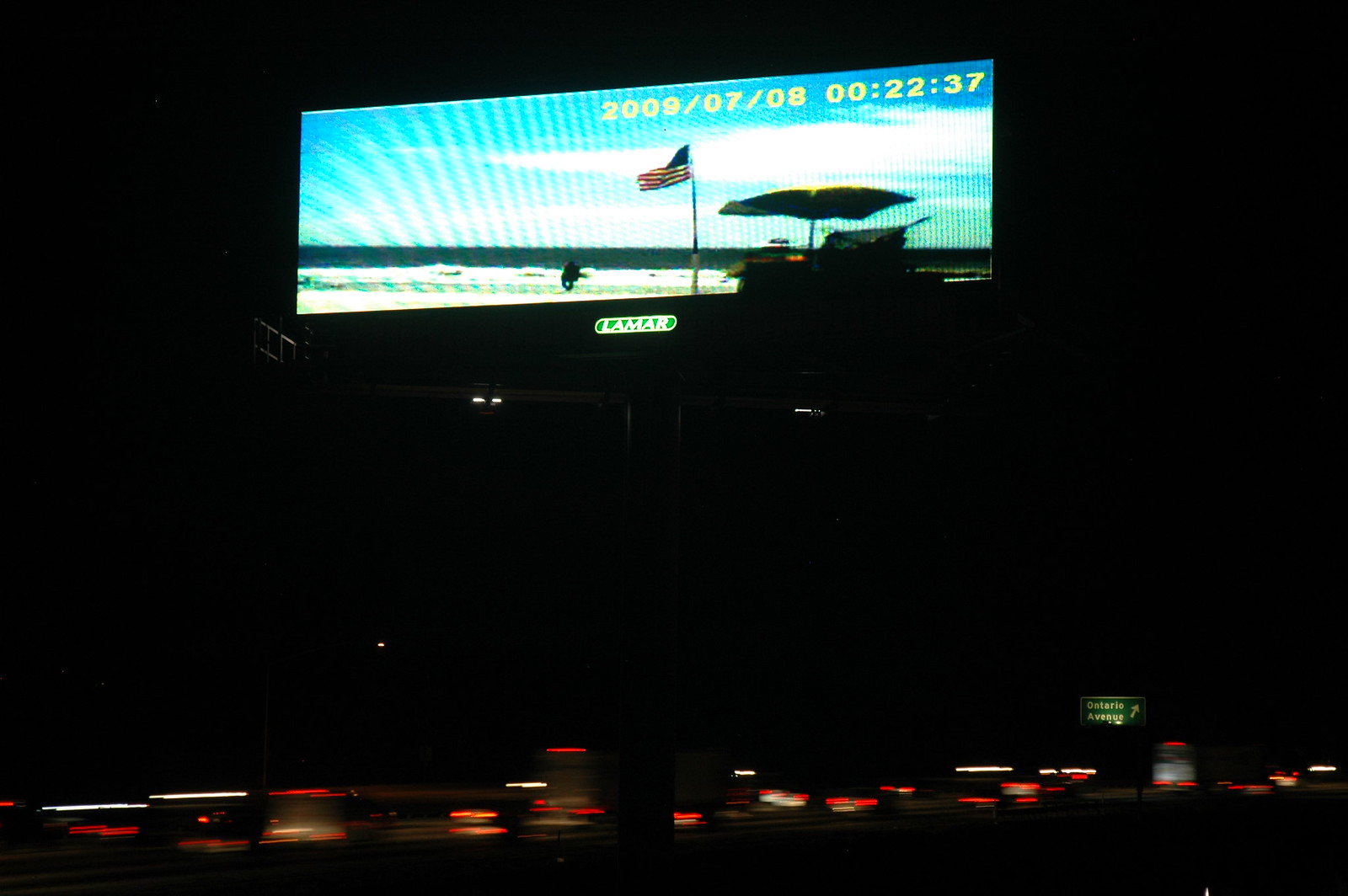This image captures a billboard situated along a busy freeway. The billboard displays a beach scene that appears heavily pixelated, giving it a nostalgic quality reminiscent of early digital photography. A date stamp on the image reads "July 8th, 2009," suggesting the photo was taken with a digital camera. Below the billboard, a stream of red taillights reveals the presence of moving traffic, indicating it's likely taken during evening hours. In the background, a sign reads "Ontario Arrivals," implying that this billboard is located near an airport in Ontario, potentially targeting incoming travelers with its beach-themed advertisement. The juxtaposition of dated technology with modern traffic and airport signage creates an intriguing blend of temporal and spatial elements in the scene.